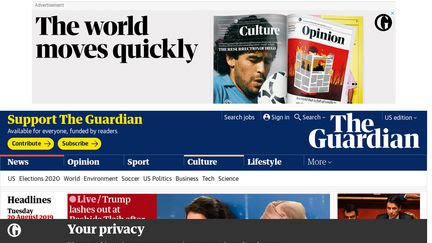In this detailed image, a person dressed in a blue shirt with black hair is prominently featured holding up a white object near their face. The object appears to be an open magazine emblazoned with the word "Culture" on one page and "Opinion" on the other. The magazine is identified as The Guardian through various visual cues. A large text reading "The Guardian" is displayed on a black background to the right. 

Other textual elements include options like "Search jobs," "Sign in," "Search," "Support The Guardian," along with prompts to "Continue or subscribe" and "Contribute or subscribe," highlighted in clickable yellow bubbles. Below this, a navigation menu lists categories such as "News," "Opinion," "Sport," "Culture," "Lifestyle," and "More."

The page also contains a section with photographs under the header "Headlines," dated Tuesday, August 20th or 29th, 2019. One headline reads, "Live: Trump lashes out at," but the text is cut off. Included in the images are partial views of people's heads, one with black hair and the other with blonde, as well as two men in what appears to be a formal setting like a courtroom.

At the bottom of the image, a black bar labeled "Your privacy" obscures part of the content, truncating the lower portion of the pictures. This extensive composition highlights both the journalistic elements of The Guardian and the detailed layout of the webpage.